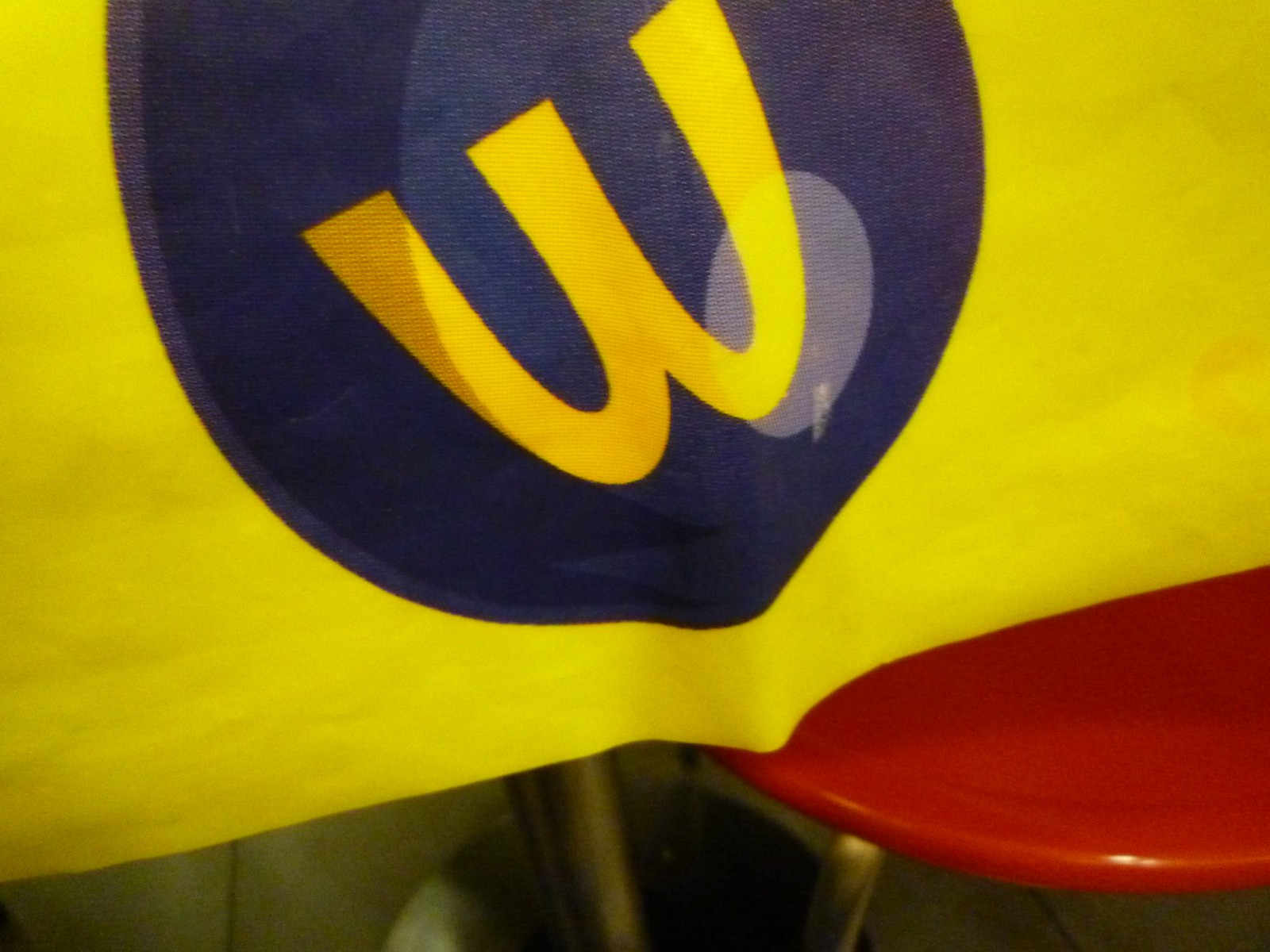This image showcases a rectangular, close-up picture of a yellow banner or fabric draped over a red stool or bench, featuring prominent silver metal legs. Dominating the yellow fabric is a large, dark navy or almost black circle. Within this circle is the iconic McDonald's golden arches logo, inverted to resemble the letter "W." Adding to the unusual visual, a smaller gray or light blue circle dips behind the upper edge of one of the inverted arches, evoking the appearance of an eye. The background of the image has blurred, grayish-brown tile flooring, enhancing the sense of depth and context in the scene.